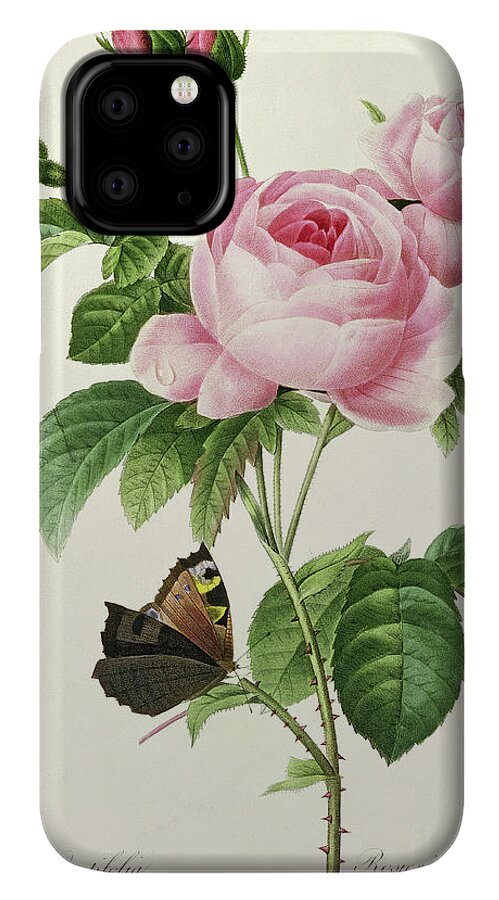The image showcases the back side of an off-white smartphone case, likely designed for an iPhone. The case features a detailed, old-fashioned botanical illustration centered around three pink roses. The upper right corner displays two roses in full bloom, while the upper left corner shows budding roses accompanied by serrated-edged green leaves. A thorny green stem extends from these flowers, splitting toward the bottom of the image. Perched on a leaf near this split is a brown butterfly adorned with black, yellow, and white splotches on its wings. In the background, behind the camera lens cutout positioned in the upper left-hand corner, additional rose buds and foliage are visible. The illustration is further detailed with delicate, spidery script at the bottom, possibly identifying the rose species as 'Rosa.' The overall design lends a charming, vintage feel to the smartphone case.